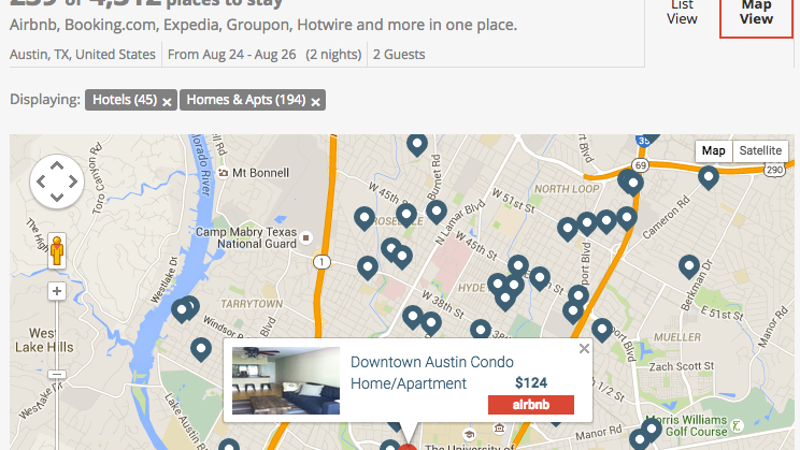This image depicts a detailed map of Austin, Texas, United States, highlighting available accommodations through platforms such as Airbnb, Booking.com, Expedia, Groupon, and Hotwire. The map is set for a stay from August 24 to August 26, accommodating two guests for two nights. Both list and map views are visible, showcasing 45 hotel options and 194 homes and apartments. Prominent locations marked on the map include Camp Mayberry, Texas National Guard, Mount Bonnell, Westlake, Windsor, Lake Austin, Westlake Hills, Dehigh, Cerro Canyon Road, Bonnet Road, Lima Boulevard, Zack Scott Street, and Moeller Road.